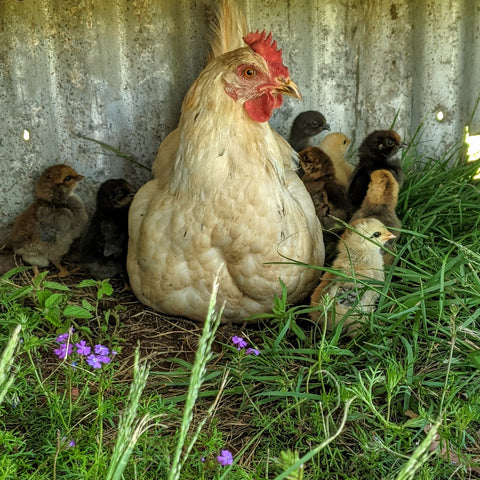This color photograph features a central white hen, plump and sitting on a patch of green grass adorned with small purple flowers. The hen's lower body starts about a third of the way up the image. She has a distinct pinkish-orange beak and a brilliant red coxcomb atop her head, with brown eyes in profile, peering to the right. Behind the hen and her chicks, there is a corrugated metal fence. To her left are two chicks: one dark brown and one black, both facing their mother. On her right are six more chicks of varied colors, from dark brown to light yellow, including a light-colored chick at the front of the photo facing away with an almost smiling expression. The grass around them also includes a mix of small purple flowers and some yellow ones, enhancing the lush, natural setting.